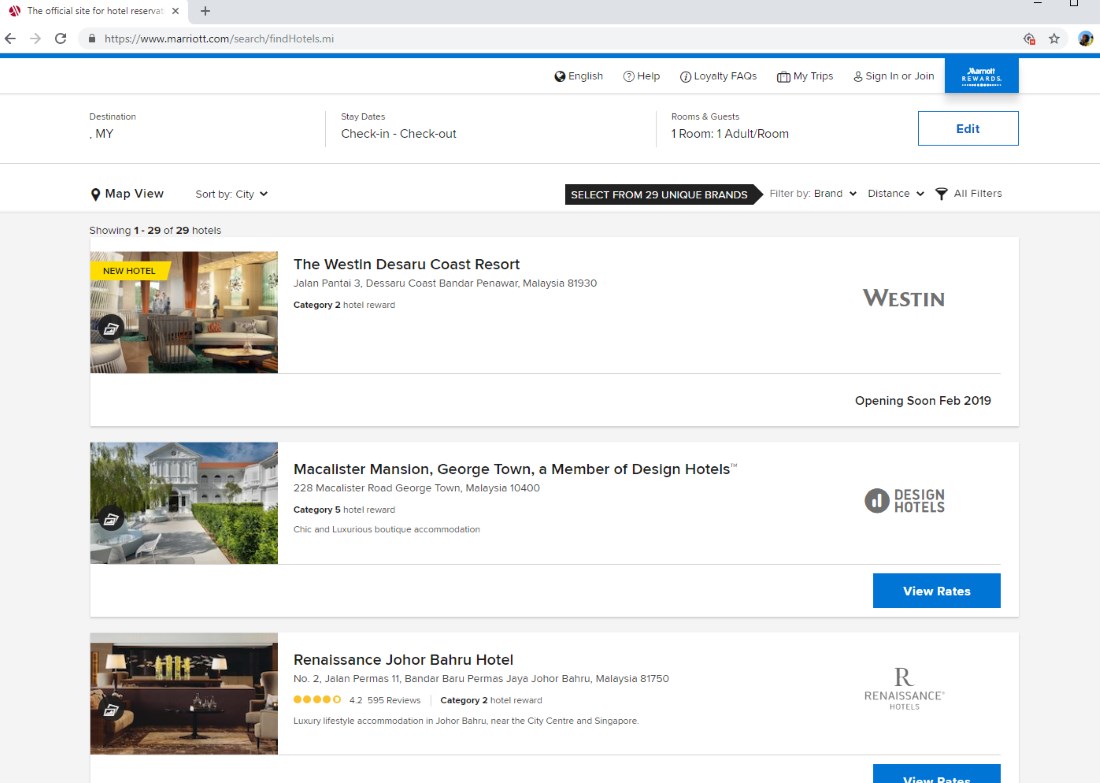This image is a landscape-mode screenshot of the Marriott website. The top left corner shows a browser tab partially reading "The official site for Hotel Reserve..." followed by a URL, "www.marriott.com/search/findhotels.mi". Below this header is a white stripe with a gray background featuring navigation options: "English," "Help," "Loyalty," "FAQs," "My Trips," "Sign In or Join," and a prominent blue button labeled "Marriott Rewards."

The next section is a search form for booking stays, displaying various input fields such as "Destination MY," "Stay Dates," "Check In," "Check Out," "Room and Guest," with a default selection of "one room, one adult," and an edit button. Additional controls for "Map View," "Sort by City," "Select from 29 Unique Brands," "Filter by Brand," "Distance," and "All Filters" are also present.

On the left side, it indicates "Showing 1 to 29 of 29 hotels," but only three are visible in the screenshot. The first hotel listed is the new "Westin Desiree Coast Resort" in Malaysia. The second listing is the "McAllister Mansion, Georgetown," a member of Design Hotels in Malaysia, followed by the "Renaissance Johar Bahru Hotel," also in Malaysia. The upper right of the screen mentions the Westin opening soon in February 2019. Each hotel listing features a "View Rates" button, with the Renaissance Hotels listing partially displaying a blue button. The page appears to be scrollable for further hotel options.